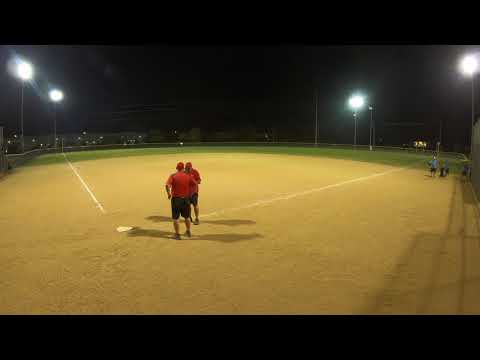This nighttime image captures a baseball field illuminated by tall dusk-to-dawn light poles against a black sky. The field's distinct V-shaped layout, with a white line marking the edges and home plate situated in the crease of the V, features a brown dirt infield and a green grass outfield in the background. At the center of the image stand two individuals clad in red shirts, black shorts, and red ball caps, possibly umpires, positioned near home plate. To the far right, along a fenced area, stand approximately four individuals, with at least two of them wearing blue shirts. The stadium lighting is prominent, with visible floodlights near the upper left corner and another set slightly further left, casting strong shadows. The image appears to be taken from behind home plate, capturing the field from this vantage point. Though difficult to discern specific details, there is also some barely visible seating in the distant background and a poorly seen scoreboard.